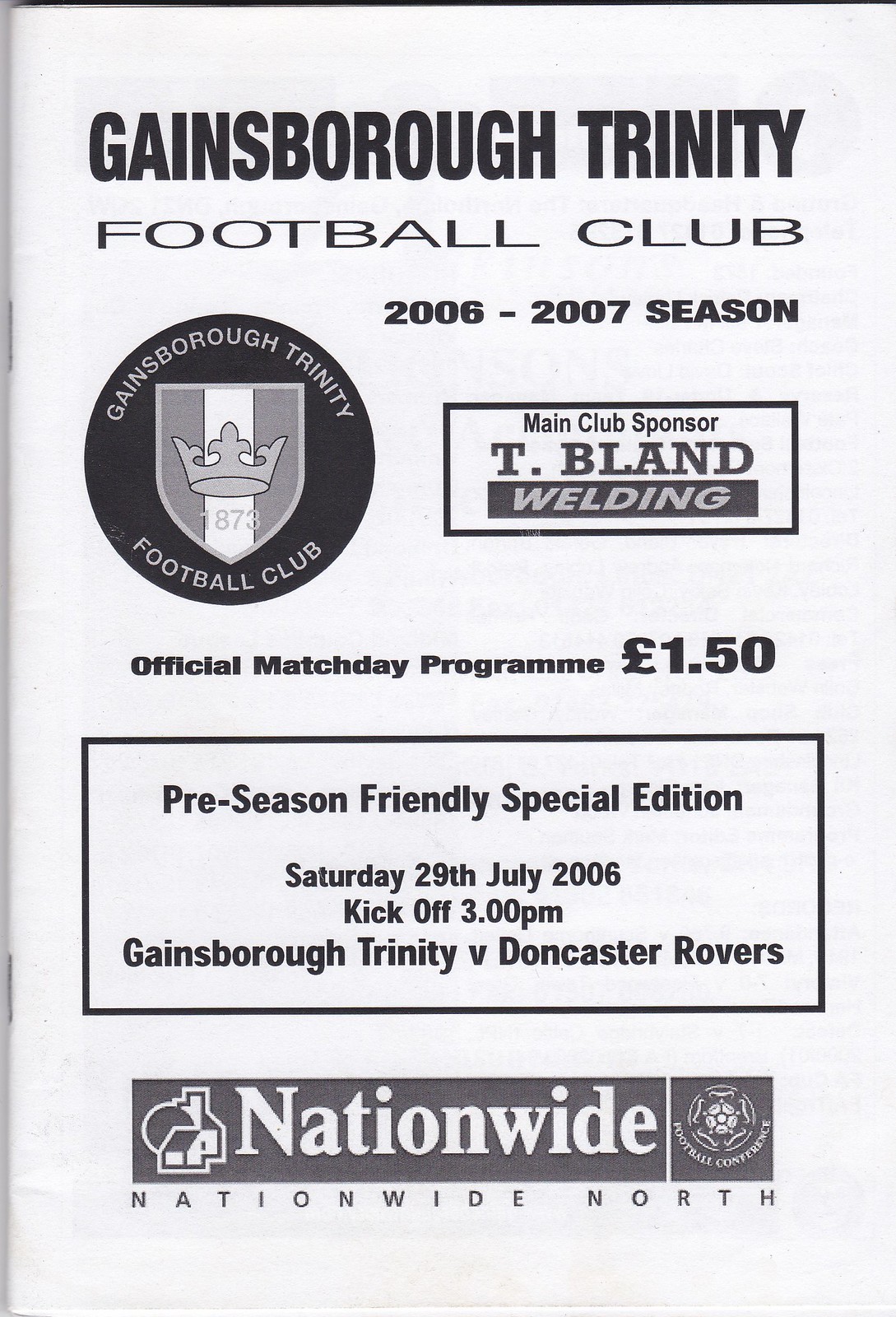This image is a detailed printed advertisement, likely appearing in a program or magazine, with a clean white or off-white background. At the top, bold black text announces "Gainsborough Trinity Football Club 2006 to 2007 Season". Below, there's an insignia within a black circle, featuring a shield and a crown, labeled "Gainsborough Trinity Football Club." To the right of this emblem, a bordered rectangle highlights the main club sponsor, "T Bland Welding". Below this sponsorship note, in smaller print, the text reads "Official Match Day Program" priced at "1.50 pounds". Further down, a larger, bordered rectangle contains the details "Preseason Friendly Special Edition Saturday 29th July 2006 Kickoff 3 p.m. Gainsborough Trinity versus Doncaster Rovers". At the bottom, in a smaller font, it mentions "Nationwide North".